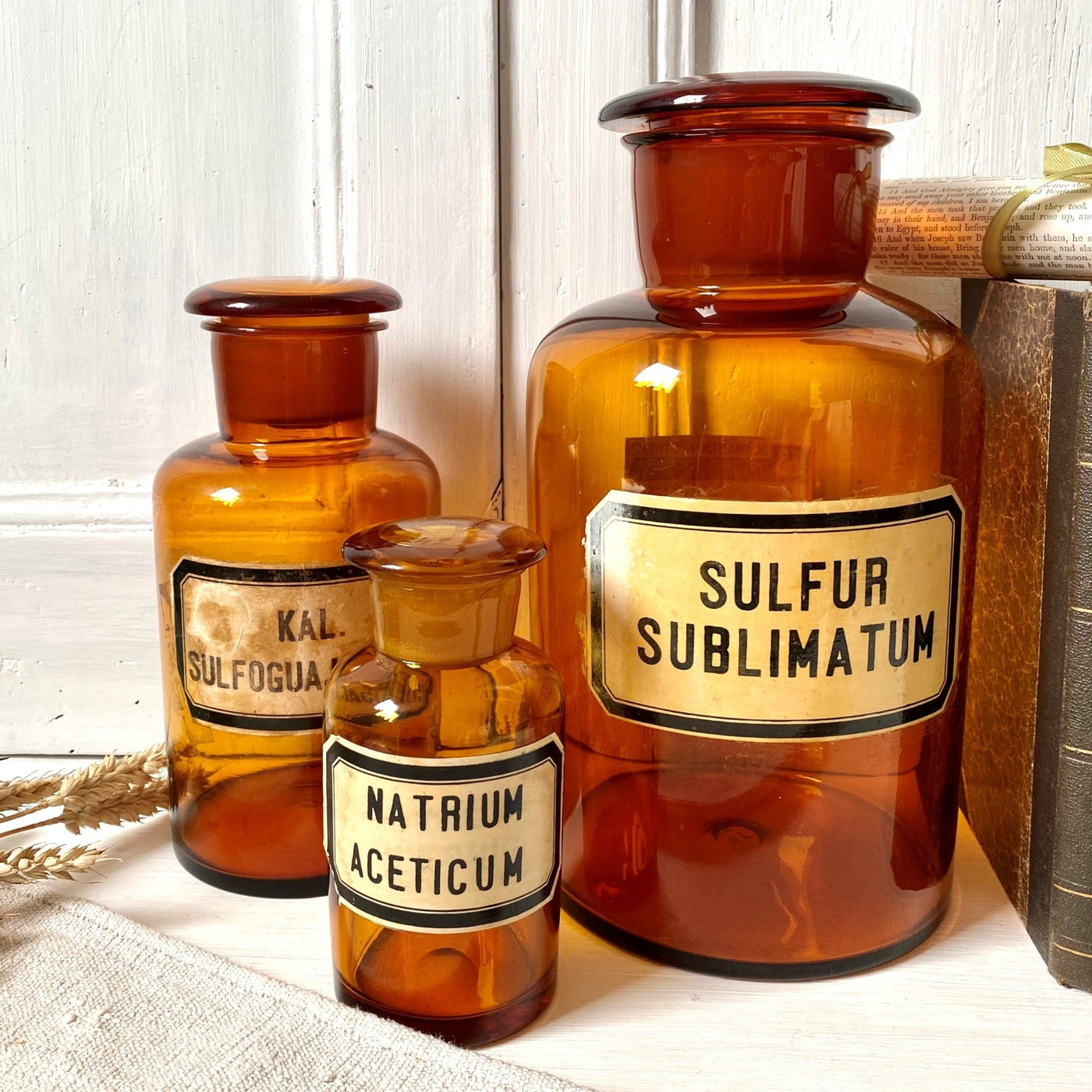The image features three transparent glass jars, each with a bronze tint, positioned on a plain white table. These jars are of different sizes, arranged from right to left in descending order, with the largest on the right. Each jar bears a label: the largest jar on the right is labeled "Sulfur Sublimatum" in black text on a red or gold label with a black outline. The medium-sized jar in the middle is partially obscured by the smallest jar, but the visible text suggests it reads "Colesulfogua-something." The smallest jar in the front bears the label "Natrium Aceticum." All jars appear to hold historical significance, possibly containing old chemicals or substances. They are set in a mostly white room, near some books, and a branch of wheat lies next to them. The scene is further complemented by a wooden window in the background.